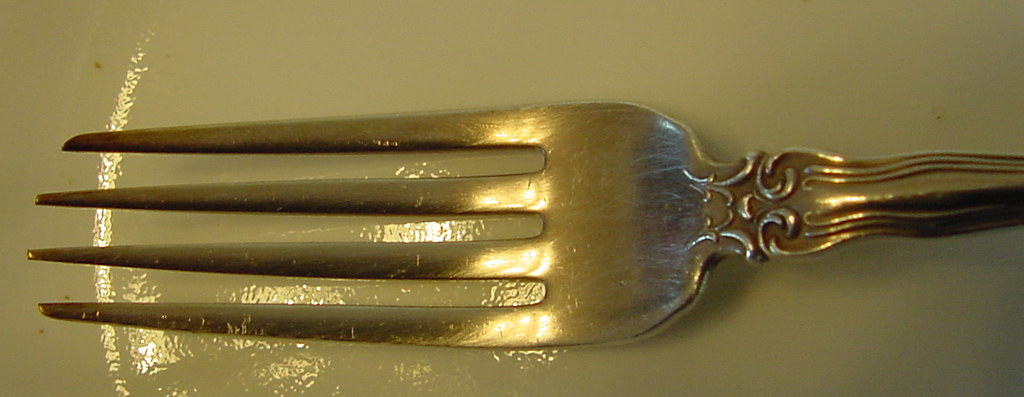The image is an extreme close-up of a fork, primarily showcasing its tines, in a landscape and very wide, narrow orientation. The fork, which appears to be made of stainless steel with a slight antiqued finish, occupies most of the frame and is positioned horizontally with its tines pointing to the left. The two central tines are longer than the outer ones. Just to the right of the tines, the fork's ornate handle is partially visible, characterized by intricate detailing with striations and swirl designs, suggesting a vintage style. The fork rests on what seems to be a ceramic plate, evidenced by the reflection forming a slight arc near the tines, indicating the plate's curvature. Both the fork and the plate exhibit subtle signs of use, such as light scratches and a speck on the plate. The background has a slightly off-green to dark green hue, providing gentle light that accentuates the metallic texture and reflective surfaces of the fork.